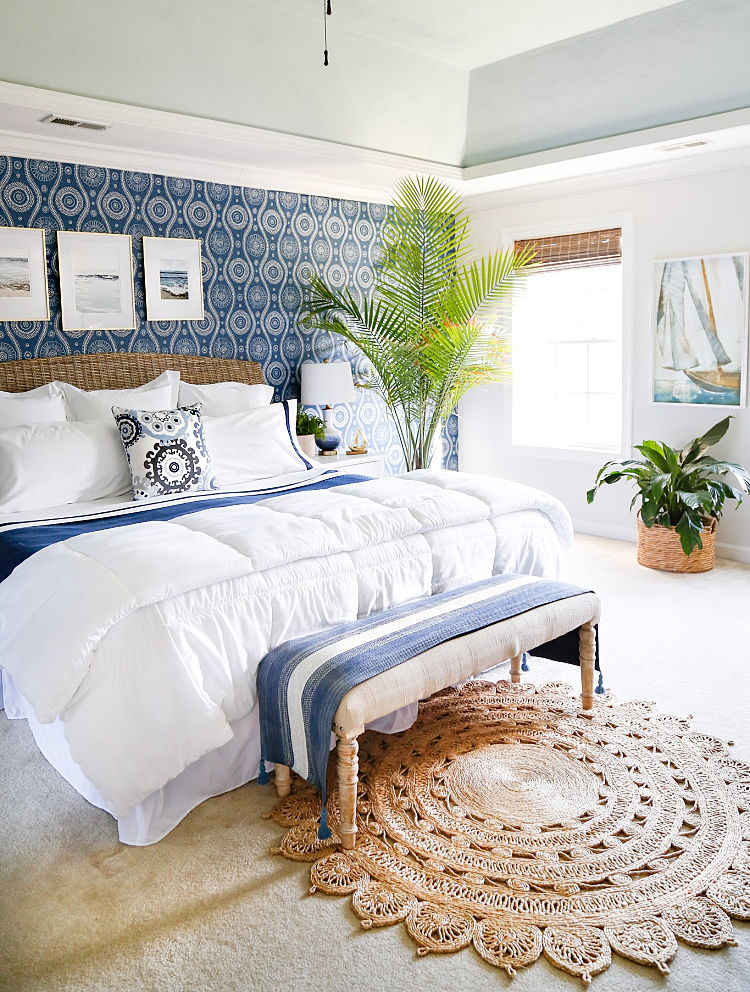This bright and airy bedroom exudes elegance and a tropical vibe. The room centers around a king-sized bed adorned with a white comforter set and decorated with a mix of white and multicolored pillows, including a distinctive blue and white decorative pillow. The headboard is made of brown wicker, complementing the overall coastal theme of the room. Behind the bed, the wall features beautiful blue and white ocean-inspired wallpaper with framed pictures of sailboats and sunny scenes.

The flooring is covered in tan carpet with a large, round, wicker-like rug adding a touch of artisan craftsmanship. At the foot of the bed, a white fabric bench with wood-spoke legs has a charming blue and white nautical blanket draped over it. The window is covered with brown woven blinds, allowing bright sunlight to flood the room, enhancing its light and inviting atmosphere. 

To the right of the bed, a sizable potted tropical plant adds a touch of greenery, while a small white table holds a lamp, providing cozy lighting for evening relaxation. Another low potted plant sits on the floor, adding to the room's natural ambiance. This serene and stylish bedroom resembles the comfort and flair of a high-end hotel or an upscale Airbnb, possibly in a tropical setting, making it a perfect retreat.